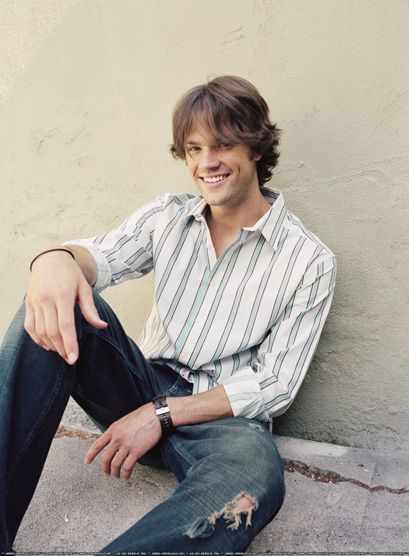This photograph features a recognizable actor, though his name is uncertain. He appears to be sitting on a cracked sidewalk outside in the daylight, leaning against a wall. The actor is dressed in a casual button-up shirt, which is partially tucked in and has rolled-up sleeves. He is wearing dark blue denim jeans that have a rip at the left knee. On his left wrist, he sports a watch, and he also has a small rope bangle. His long, dirty brown hair, parted in the middle, cascades past his collar with some strands covering his eye. The actor has a friendly smile showing his white teeth as he looks directly at the camera. His pose is relaxed with one knee up, arm resting on it, while the other leg is stretched out on the ground and his other arm rests near his crotch. The visible colors in the image include light tan, white with grey stripes, black, and off-white or grey for the sidewalk.